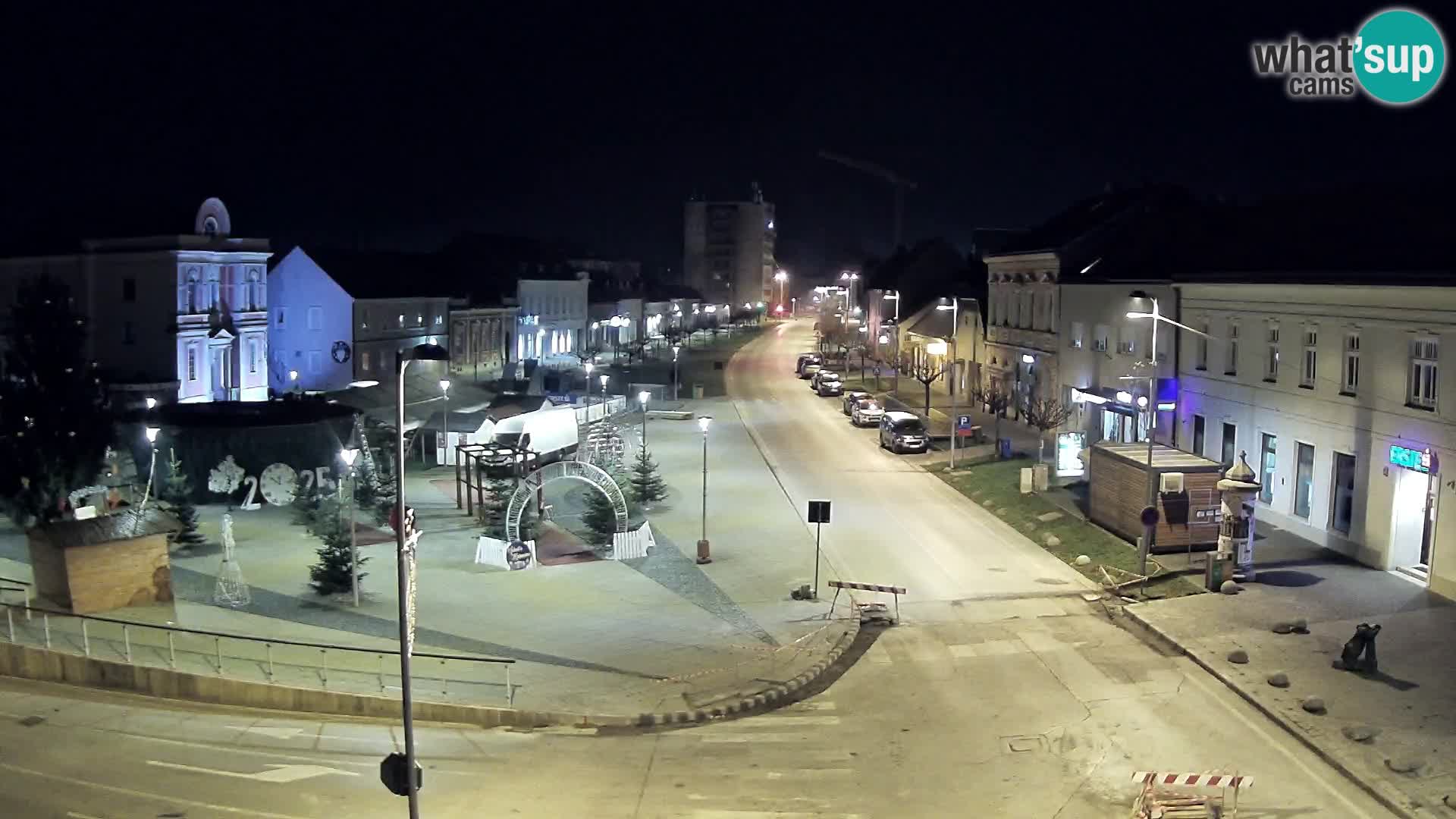This is a detailed nighttime photograph of a city street illuminated by streetlights. The street, appearing light beige despite being asphalt, runs diagonally from the lower left to the upper right, intersecting with another street that crosses from left to right near the bottom and continues straight through the middle. The streets feature two prominent crosswalks marked with visible tar lines. Numerous buildings line the street, with structures on the right being mostly two stories high, featuring white facades and windows, some of which are lit. Towards the far end, a taller building dominates the background. Cars are parked along the right side of the street, including one near the curve with its bright white lights shining and a door ajar. The skyline is pitch black, indicating it is nighttime. Additionally, a string of buildings with varying wall colors, including white and darker brown, stretches along the street. In the upper right corner of the image, a green circle enclosing the word "SUP" is displayed, flanked by the words "WHAT'S UP" above and "CAMS" below, indicating a dash cam capture. The surroundings show a small, unusual business district with no prominent sidewalks, just flat areas interspersed with grass and boulders.